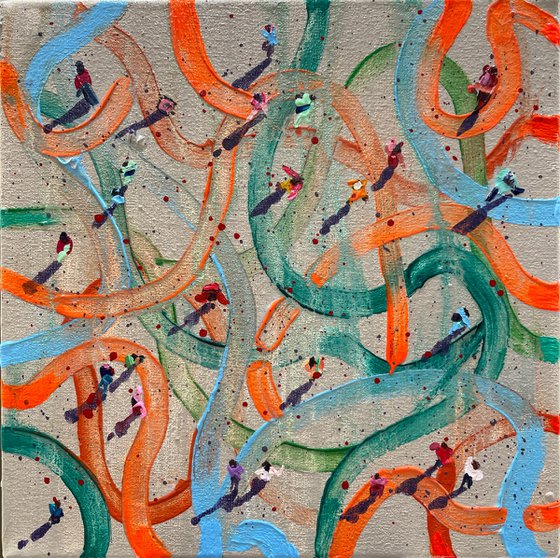This modern abstract painting on a square, textured beige canvas is a vibrant explosion of color and movement. The artwork is dominated by sinuous, snake-like streams of paint that appear to have been applied with a finger, spreading as if in a finger-painting technique. These narrow, curving streaks of paint, with thick, heavily layered edges, meander across the canvas in all directions—upwards, downwards, and diagonally—creating a dynamic, flowing composition. The colors of the swirling lines range from various shades of teal and forest green to vibrant light and dark oranges, with some light blue interspersed among them. Adding to this complex interplay of colors are additional linear splatters in predominantly blue, red, and purple hues. The purple splatters, in particular, feature intricate tips with touches of white, red, and purple, enhancing the multi-dimensional texture and visual interest of the painting. This non-representational work captures a sense of chaotic energy and movement, leaving an impression of vibrant, tactile complexity.